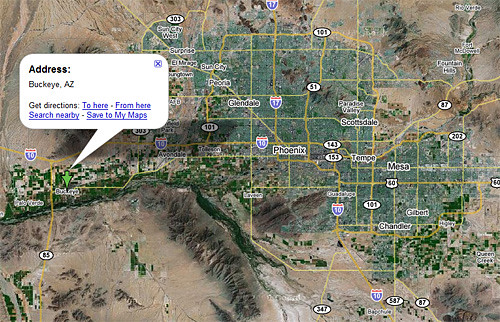This highly detailed computerized map provides an intricate view of the Phoenix metropolitan area. At the center of the map is Phoenix, surrounded by notable neighboring cities such as Mesa, Tempe, Chandler, Gilbert, Scottsdale, Paradise Valley, Glendale, Peoria, Sun City, and Avondale, all of which are clearly labeled. The major freeways that traverse the area, including I-10 and I-17, are prominently marked, alongside additional significant routes like SR-51, Loop 101, US-60, SR-143, and SR-153, showcasing the extensive highway network.

The map artfully distinguishes the urban landscape with green shading to highlight the central city area of Phoenix and its surrounding urban hubs, contrasting with the vast desert that envelops the region. A specific point of interest is marked with a green arrow, directing attention to Buckeye, Arizona, with an accompanying pop-out note that further emphasizes this location. The thorough labeling and visual markers provide a comprehensive understanding of the geography and infrastructure of the Phoenix area.